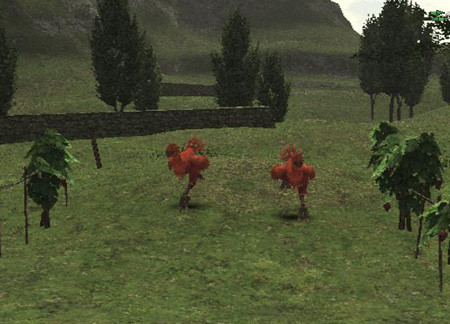The image is a computer-generated landscape scene resembling a digital painting or game graphic. In the foreground, there is an expansive field of green grass stretching into the distance. Dominating the background is a large, sharply inclined green hill that extends off the top of the screen. Near the center of the image, two large, orange, ostrich-like birds—mistakenly identified as chickens by some—are running towards the observer with red combs and long beaks. Flanking these birds are two stylized, digitized trees with a somewhat artificial appearance. Beyond the birds and trees is a low stone wall, behind which stands a more realistic grove of short, pointed trees, adding depth to the scene.